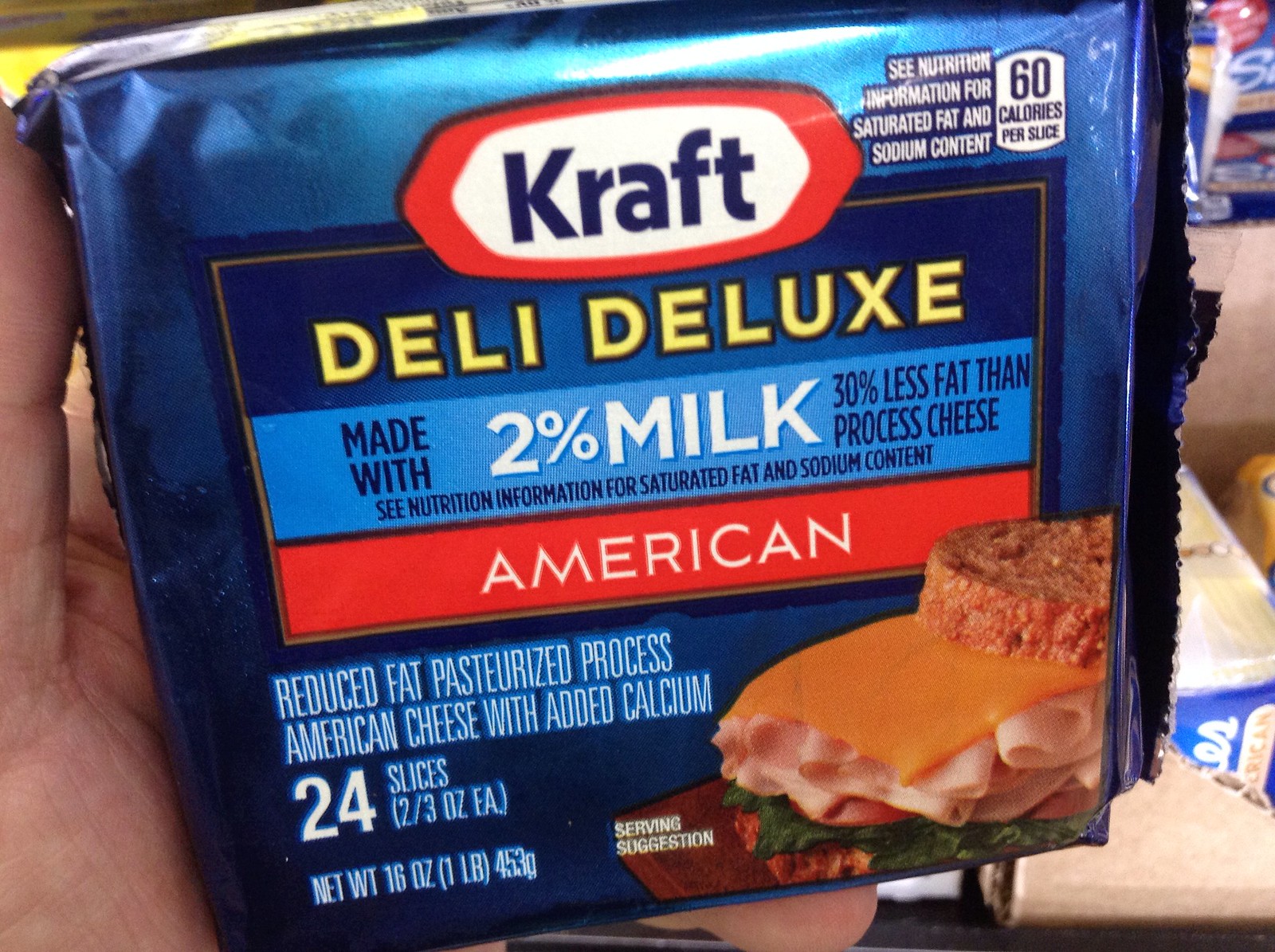The image features a package of Kraft Deli Deluxe American Cheese. A left hand prominently holds the blue packaging, while in the background, there appears to be additional cardboard packaging, likely containing more cheese. The central blue package showcases a red and white Kraft logo. Below the logo, text indicates, "See nutrition information for saturated fat and sodium content," and mentions that each slice contains 60 calories.

Further details on the packaging include:
- The product name "Deli Deluxe" in a blue rectangle.
- A light blue rectangle stating, "Made with 2% Milk, 30% less fat than processed cheese. See nutrition information for saturated fat and sodium content."

On the gray rectangle, the right side reads “American,” specifying the cheese type. Additional information at the bottom describes the cheese as "Reduced fat, pasteurized processed American cheese with added calcium." The package contains 24 slices, each approximately 0.75 ounces, totaling a net weight of 16 ounces (1 pound, 430 grams).

There is a serving suggestion image featuring a sandwich with layers consisting of a red tomato slice on top, followed by the cheese, several layers of deli meats, and a bed of lettuce.